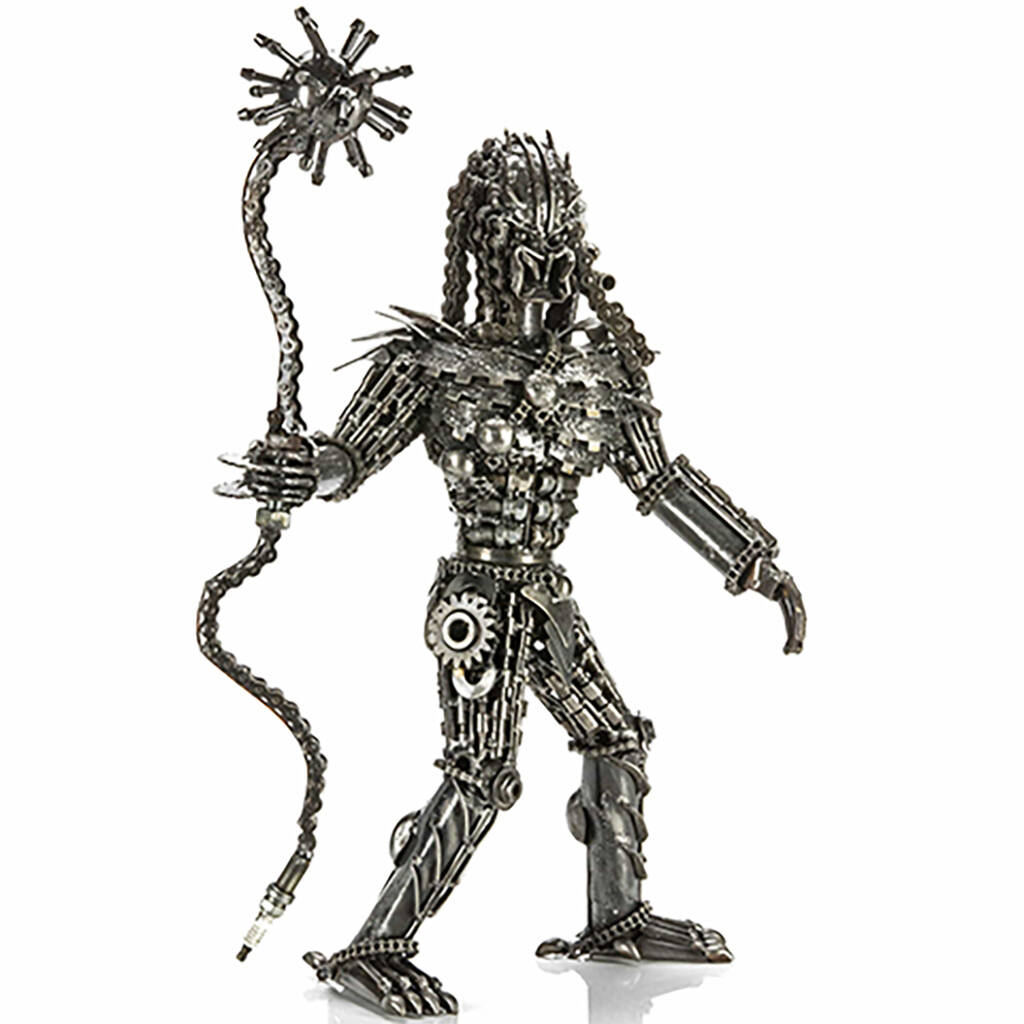In the center of a square image with a light, pale grayish-blue background, stands a meticulously detailed figurine, measuring approximately 6 inches in height and width, resembling a mechanical alien predator from the Predator series. This statue, forged from silver metalwork, features a large, bulbous head adorned with chain-like dreadlocks and a square mouth flaring open at the corners with fangs extending from four sides. Small beady eyes add an ominous touch to its menacing look. The predator, slightly leaning forward and walking to the right, showcases gears at its hip joints and several metallic components, including armor, giving it a robust, mechanical appearance. Its right hand grips a menacing weapon—a long, snake-like metal tube with numerous chain links transitioning into a spiked mace ball. This ball and chain extends towards the left side of the image while the predator's left arm dangles loosely by its side. Its sturdy feet, firmly planted on a reflective white surface, enhance the action-figure-esque style of this striking metallic ornament.